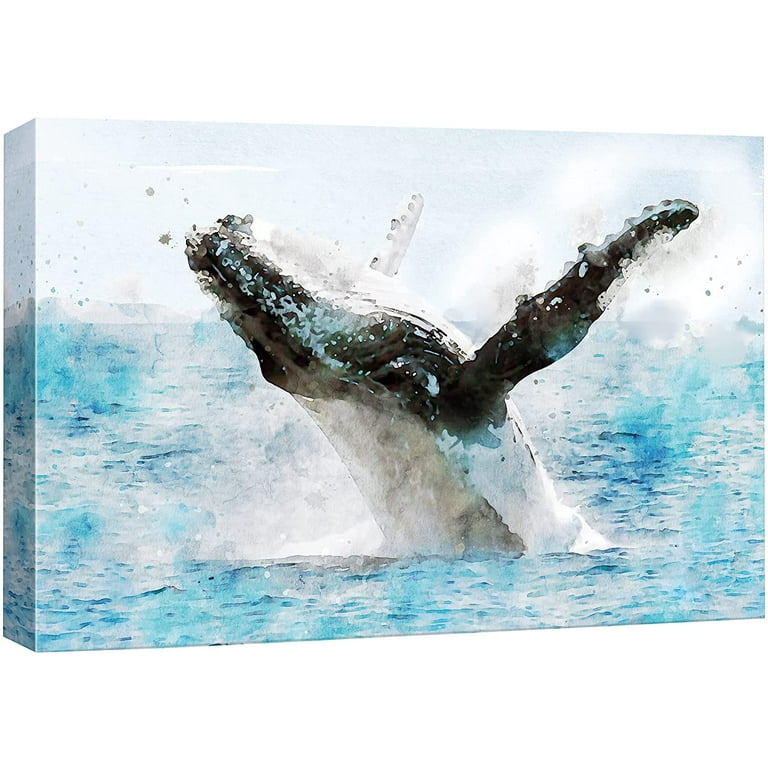This captivating piece of canvas art presents a three-dimensional, abstract watercolor depiction of a killer whale in mid-jump. Centrally positioned, the black and white whale is arching backward, its underbelly facing up. Its curved body and spread fins create the impression of dynamic motion. The whale's head is angled toward the upper left corner of the canvas, with one fin extending to the upper right and the other pointing toward the middle of the top edge. The canvas is edged, and the pale blue sky in the background contrasts softly with the vivid blue and white ocean surrounding the whale. In the distance, faint mountain shapes emerge, adding depth to the scenery. The background of this image is entirely white, emphasizing the artwork and allowing viewers to see the left edge of the canvas vividly. No text accompanies the image, letting the majestic portrayal speak for itself.